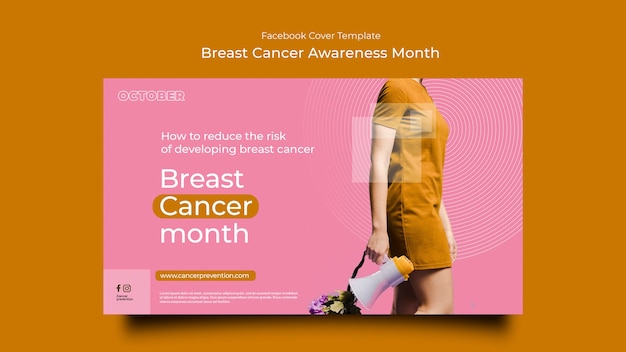The image features a burnt orange background, providing a subdued yet warm canvas. At the top, in white font, the text reads "Facebook Cover Template - Breast Cancer Awareness Month." A prominent pink square overlays the orange backdrop, and within this pink section, the word "October" is written in the upper left corner.

A woman is depicted in a side profile, holding flowers in one hand and a megaphone in the other. She is wearing a dress that matches the burnt orange of the background. Overlaying the pink box, the title "How to Reduce the Risk of Developing Breast Cancer" is displayed alongside "Breast Cancer Month" and the website "www.cancerprevention.com."

In the bottom left corner of the image, logos for Facebook and Instagram are visible. Additional white text is present at the very bottom, likely containing further information about the website or Breast Cancer Awareness Month, although it is too small to read.